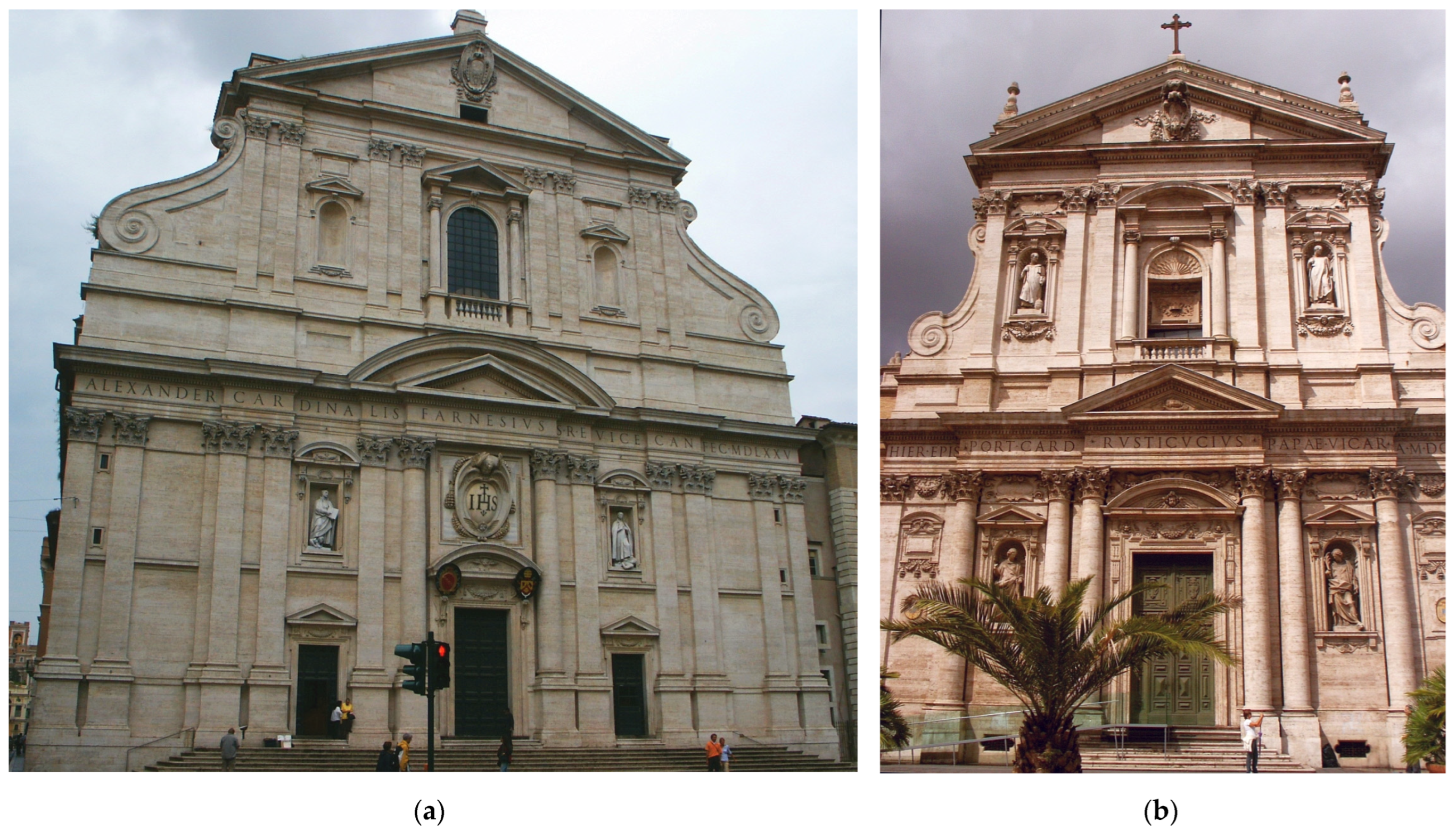This image showcases two side-by-side Baroque churches from Italy, labeled A on the left and B on the right. Both buildings share a symmetrical architectural design with rectangular and circular columns, as well as triangular pediments. Church A, constructed with beige-colored stone, features a more expansive facade, including a stoplight and steps leading up to the entrance. The front of Church A displays intricate engravings: "IHS" prominently under a U-shaped window at the top and inscriptions that read "Alexander Cardinalis Phanevas Grievous Can..." partially visible under a balcony. Statues of women adorn the window cutouts above the entrance. The building has a distinct swirled, angled design leading to its roof.

Church B, in a lighter color palette, mirrors the design of Church A but with slight differences. This church has a palm tree in front and a set of statues positioned to the sides of its door, with another set flanking the windows on the top floor. Unlike Church A, Church B features a cross atop its structure. Both buildings exude grandeur, bathed in the Baroque style, with subtle differences that make each one unique. There are a few people scattered in the scene, enhancing the scale and magnificence of these imposing structures.